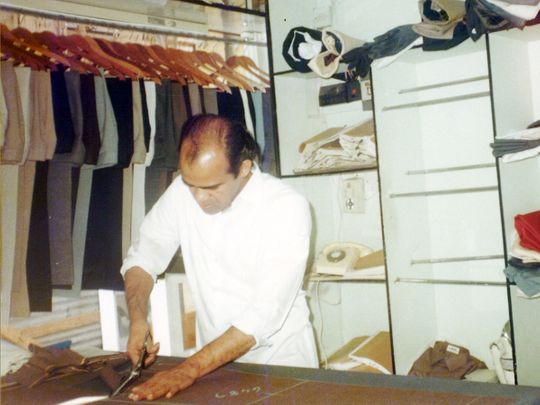The photograph depicts a man in a white, long-sleeve shirt with the sleeves rolled up, working in what appears to be a tailor's workshop. He is holding a pair of scissors and is in the process of cutting a brown piece of fabric, which has gray markings that might be cut lines for stitching. The setting is busy with numerous details suggesting a clothing-making environment: to his left, several pairs of pants and a wide range of colored, formal shirts—including shades of beige, brown, black, light gray, bluish hues, pink, light purple, and light green—hang on hangers. Behind him, white shelving holds additional shirts and a white telephone, along with rolls of fabric on the top shelf. The overall impression is that he is diligently engaged in his craft, surrounded by the tools and materials of his trade.